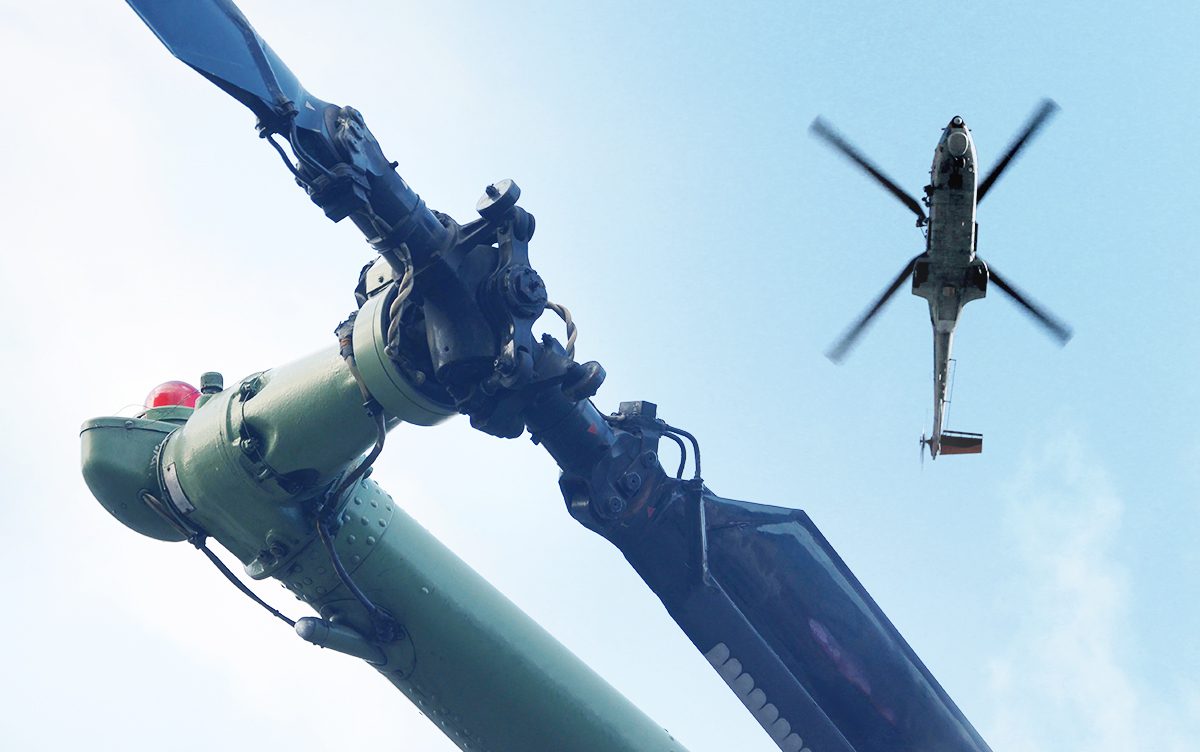The image showcases a dynamic aerial scene featuring two distinct helicopter components. In the upper right corner, a silver-gray helicopter is in flight, captured from below against a backdrop of a blue sky adorned with a few clouds. The helicopter's four main rotor blades are in motion, creating a blurry effect. Dominating the lower left corner of the image is the back rotor assembly of another helicopter, characterized by its green arm and two stationary black blades. A red flashing light is visible at the tip of the green arm, contrasting sharply against its surroundings. This detailed composition juxtaposes the active flight of the upper helicopter with the grounded presence of the lower rotor, providing a unique perspective of aerial technology in action.